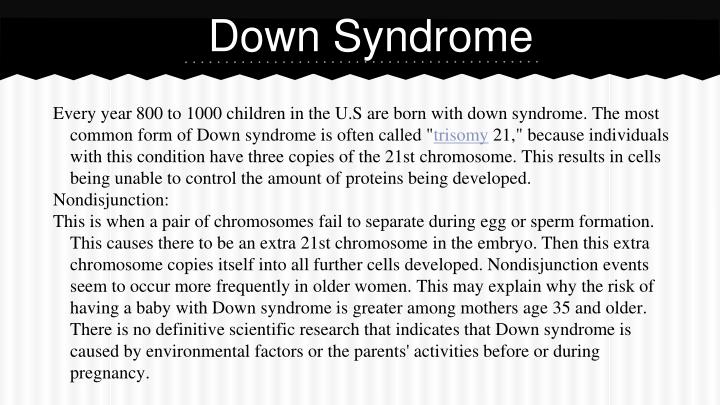This image is a screen capture of a digital document concerning Down Syndrome. At the very top, it features a black background with white text that reads "Down Syndrome," accompanied by dots underneath. Below this, a decorative pyramid border separates the black header from the main body of the text. The main section of the document has a white and gray vertical striped background with extensive information in black text.

The text discusses that each year, between 1,800 and 1,000 children in the U.S. are born with Down Syndrome. The document explains that the most common form of Down Syndrome is Trisomy 21, named because individuals with this condition have three copies of the 21st chromosome. This chromosomal anomaly prevents cells from regulating protein production correctly.

It further elaborates on the concept of "Non-disjunction," a process where a pair of chromosomes fails to separate during the formation of egg or sperm cells, leading to an extra 21st chromosome in the embryo. This extra chromosome is then replicated in every subsequent cell. The document notes that non-disjunction events occur more frequently in older women, which may explain the increased risk of Down Syndrome in babies born to mothers aged 35 and older.

The text concludes by stating that there is no conclusive scientific evidence linking Down Syndrome to environmental factors or the activities of parents before or during pregnancy.